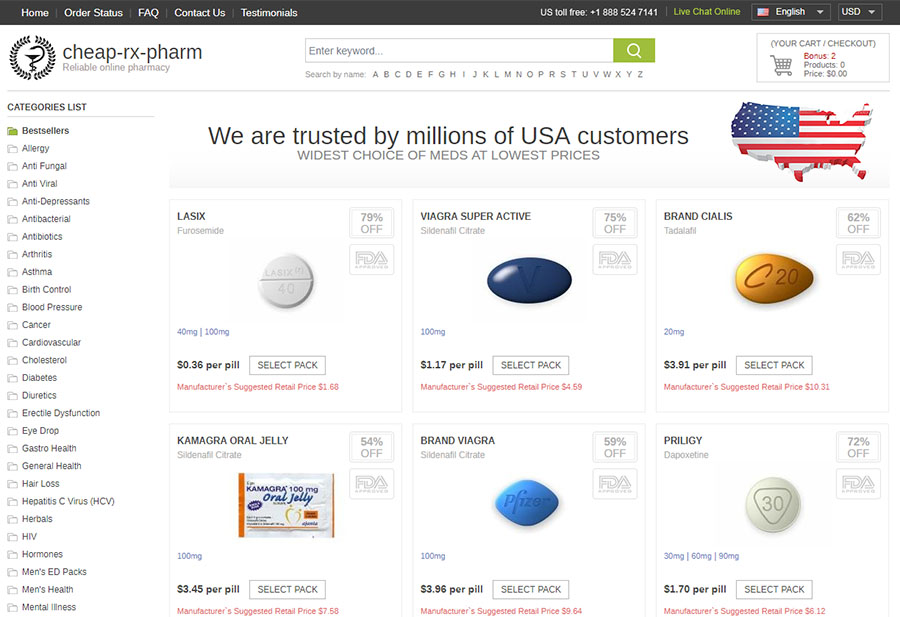The web page features a sleek design with a prominent black rectangular header running horizontally across the top. The header contains essential navigation links in white lettering, including "Home," "Order Status," "FAQ," "Contact Us," "Testimonials," and "U.S. Toll-Free" with an accompanying phone number. A green "Live Chat Online" button stands out beside language and currency options, "English" and "U.S.D." respectively, accompanied by an American flag icon preceding the language selection.

Below the header, the site prominently displays the title "Chief R.X. Farm" in black text against a white background. Adjacent to this title is a search bar labeled "Enter keyword," paired with a green "Search" button. Additionally, a shopping cart icon labeled "Cart/Checkout" summarizes the user's cart contents, mentioning a bonus and listing the product names and prices.

The center of the page features a bold statement: "We are trusted by millions of U.S. customers, widest choice of meds at lowest prices," superimposed over a U.S.-shaped American flag graphic.

On the left-hand side, a vertical column lists product categories under "Categories List," including popular best sellers organized alphabetically from allergies to hair loss. These categories encompass various medical conditions such as allergies, antifungal, arthritis, birth control, blood pressure, cancer, eye health, gastro health, and hair loss.

The main content section of the page is structured with two columns of product visuals. Each product entry displays an image either of the pill or its packaging. The first column showcases:
1. "LASIK," featuring a white pill divided by a line, labeled "LASIK" with "40" below.
2. "Camargo Oral Gel" accompanied by an image of its packaging.
3. "Viagra," presented as an oval-shaped blue pill.
   
The second column highlights:
1. "Brand Viagra," a diamond-shaped blue pill with "Pfizer" inscribed.
2. "Brand CIALIS," depicted as a sideways teardrop-shaped pill with "C 20" on it.
3. "Cryology," a circular pill with a triangle and the number "30" inscribed.

Each product entry is detailed with its name and a representative image, providing a clear visual reference for online shoppers.